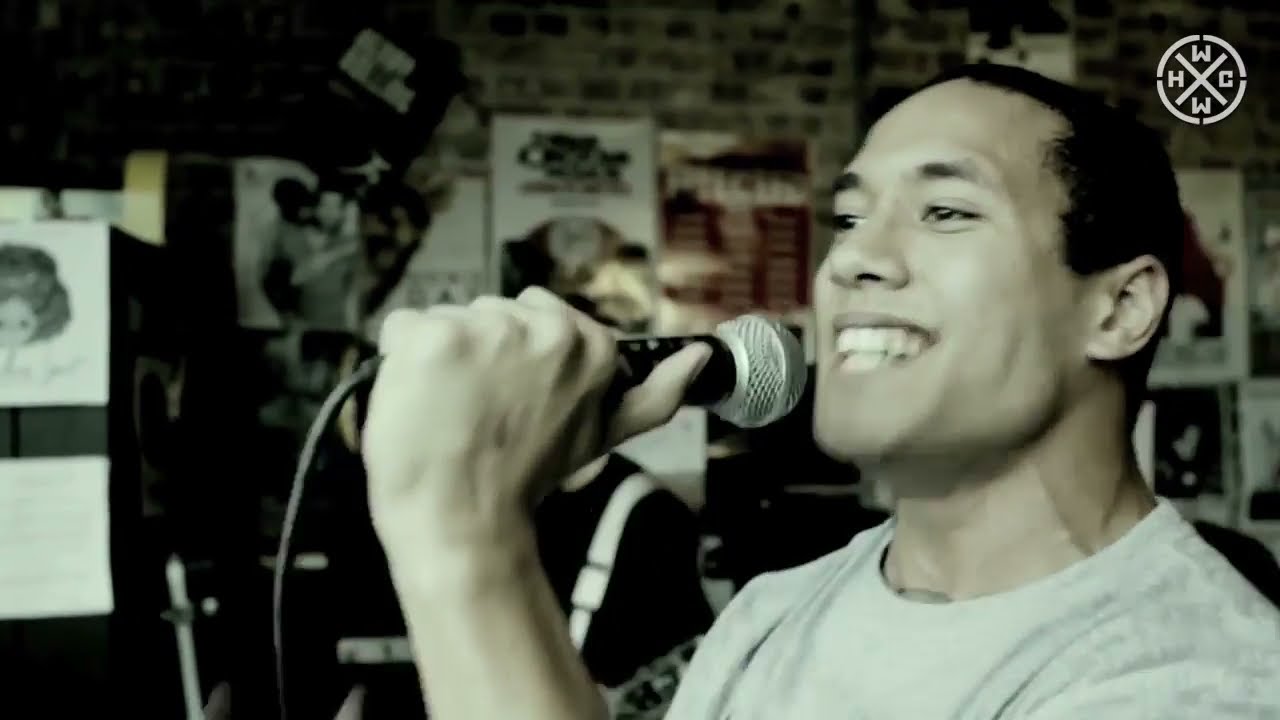The photograph captures a young white man in his 20s intently playing a drum set in a room with beige off-white walls. The room’s corner walls are adorned with an eclectic range of artwork, magazine covers, posters, and possibly vinyl album covers. Dominant among them is a bright blue poster on the right side. The drum set, positioned centrally at the bottom part of the image, comprises four drums with white surfaces and silver metal linings; one drum has a distinct red body. The setup includes three golden cymbals—two mounted to the left and above the drums, and one to the right in front.

The drummer, clad in a gray T-shirt featuring an orange, black, and white logo with text, and black pants, has dark hair with long bangs, a black round earring, and possibly a tattoo on his right arm. A black necklace adorns his neck, adding to his casual yet expressive persona. His left hand appears in motion, striking the drums with drumsticks, indicating he is actively playing. The photo exhibits a nostalgic, slightly faded quality reminiscent of the 70s or 80s, enhancing its vintage feel.